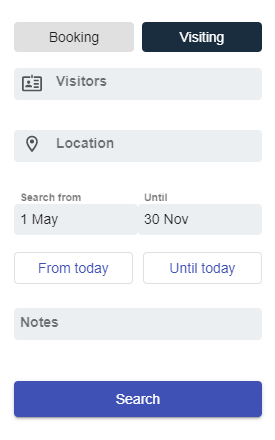This image is a screenshot of a booking page, specifically the 'Visiting' section, which is currently selected as indicated by a dark blue box while the 'Booking' option is represented by a gray box, highlighting the active tab. Directly underneath, there's a gray bar featuring an ID badge icon next to the word "Visitors." Below this is another gray input field adorned with a navigation pin icon labeled "Location."

Further down, a gray bar is prominently displayed with the text "Search from and until" on top. Within this section, the gray input box includes the placeholder text "1 May - 30 November." Following this, there are two white boxes, each outlined with thin gray lines: the first box displays "from today" in blue font, and the second box shows "until today" in the same blue font.

Lower on the page, there is another gray box designated for inputting notes, and at the very bottom, a blue "Search" button is prominently displayed, ready for user interaction.